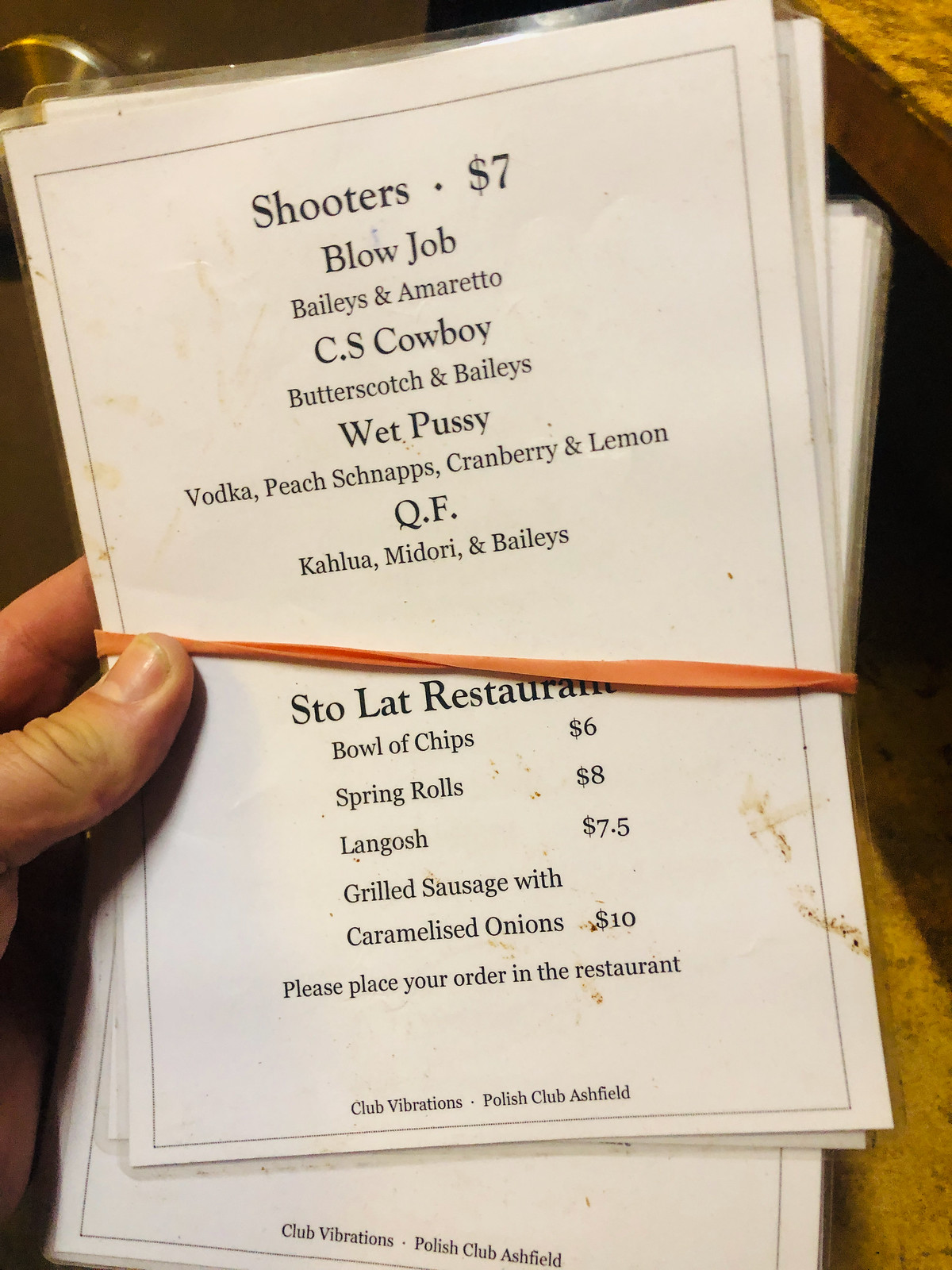This photograph features a hand holding a slightly disheveled stack of A5 menus. These menus, associated with Club Vibrations at the Polish Club in Ashfield, USA, detail both drink and snack options, and the prices are listed in dollars. The approximately seven or eight menus are partially fanned out, reminiscent of a splayed deck of cards, and secured with a single red elastic band, although the top few menus have slipped slightly to the left.

Highlighted drink offerings include a variety of shooters priced at $7 each: 
1. Blowjob – Baileys and Amaretto
2. CS Cowboy – Butterscotch and Baileys
3. Wet Pussy – Vodka, Peach Schnapps, Cranberry, and Lemon
4. QF – Kahlua, Midori, and Baileys

The Stowlat Restaurant’s snack menu lists items such as a bowl of chips, spring rolls, langosh, and grilled sausage with caramelized onions. Patrons are advised to place their orders directly at the restaurant.